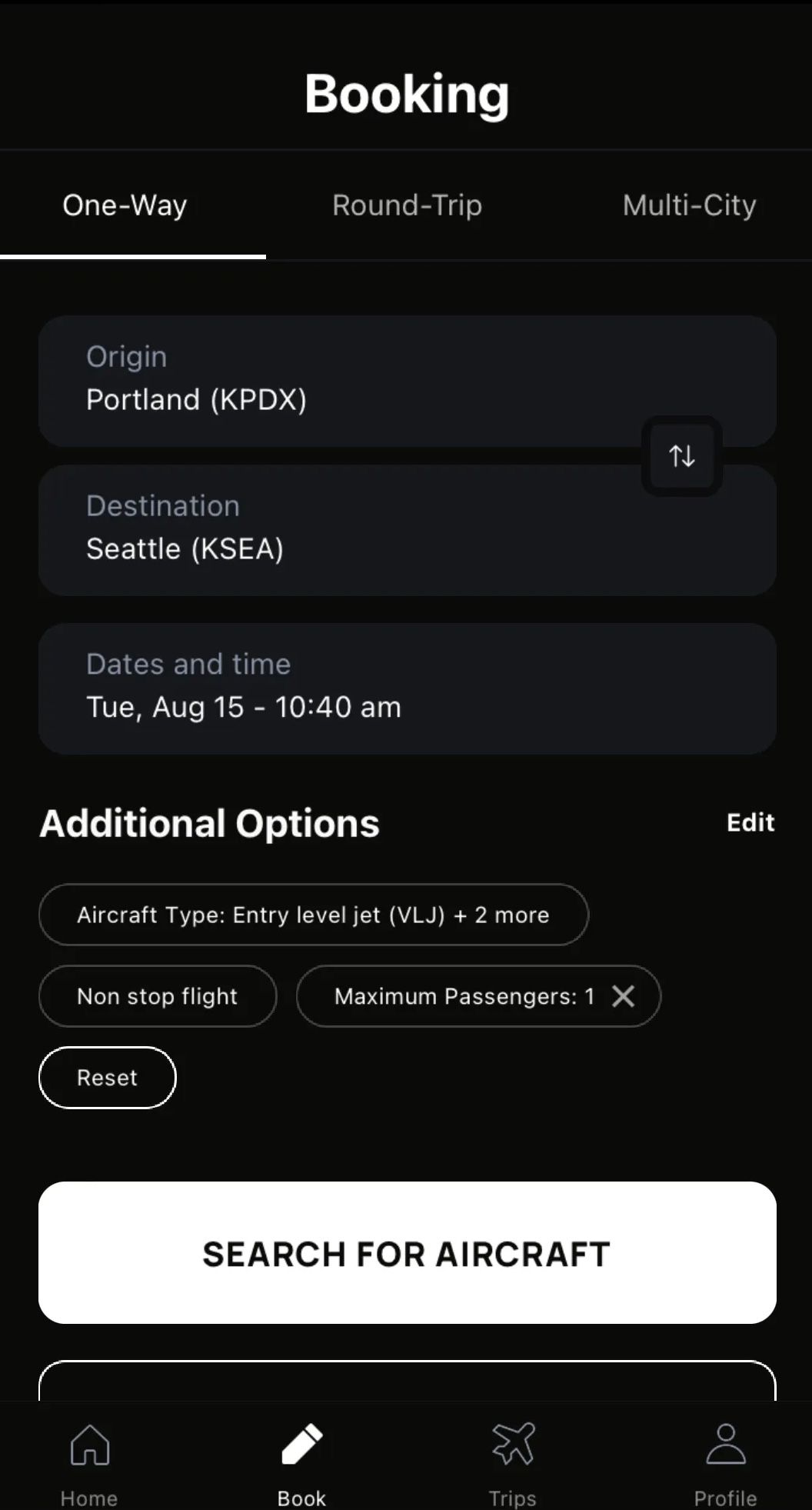The image depicts a sleek, dark-mode flight booking interface. The background is black, providing a contrasting backdrop for the primary elements which are highlighted in white. The user is currently focused on booking a "One-way" flight, evidenced by the bold white selection with a thick underline.

Three booking options are available: "One-way," "Round-trip," and "Multi-city," with "One-way" prominently selected. Below this, the interface displays sections for the origin and destination of the flight. The text for the origin is in gray, indicating it’s not currently the active selection, while "Portland" is clearly marked as the destination. There is also an option to interchange the origin and destination easily.

The interface shows a date and time of departure: "Tuesday, August 15th at 10:40 AM." Additionally, there is a section for "Additional options" which is highlighted in bold white text. To the right, an "Edit" button allows for modifications. Users can select aircraft type from several options including "Entry Level Jet," among two others. They can also specify preferences for non-stop flights and adjust the maximum number of passengers. A "Reset" button allows users to clear their selections.

At the bottom, a prominent white button with black text invites the user to "Search for Aircraft." Navigation options include "Home," "Book," "Trips," and "Profile," with "Book" being more pronounced, indicating it is the current section.

Overall, the interface is designed for ease of use, with clear, easy-to-read options and an intuitive layout for booking flights.